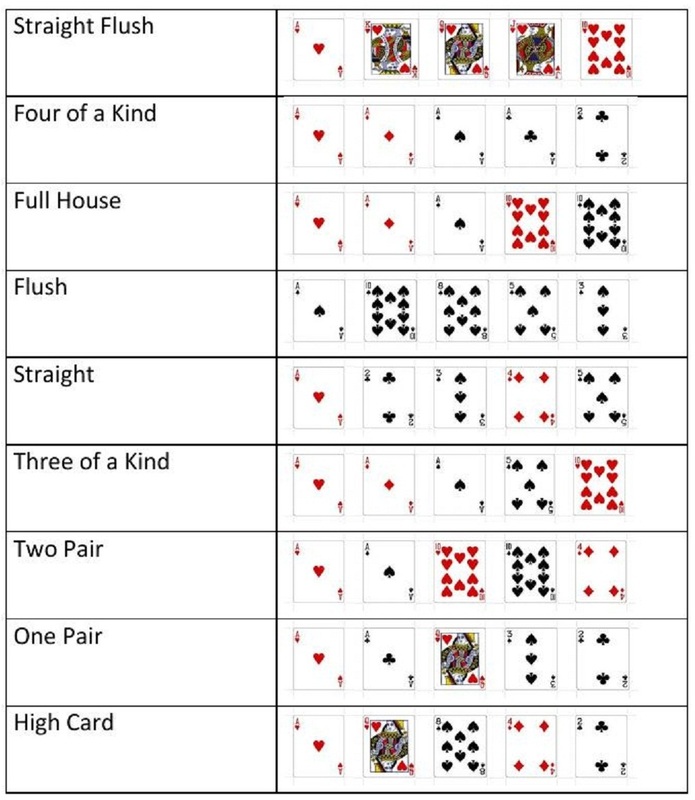This image is a detailed diagram illustrating various poker hands. The diagram is organized into two columns and ten rows. The left column lists the names of the poker hands, while the right column provides visual illustrations of each hand.

- **Top row, labeled "Straight Flush":** Features a sequence of cards all in hearts – Ace, King, Queen, Jack, and Ten.
- **Second row, labeled "Four of a Kind":** Depicts four Aces along with a Two of Clubs.
- **Third row, labeled "Full House":** Shows three Aces (hearts, diamonds, clubs) paired with two Tens (hearts and spades).
- **Fourth row, labeled "Flush":** Displays five spades: Ace, Ten, Six, Five, and Three.
- **Fifth row, labeled "Straight":** Contains a mixed suit sequence of Ace of Hearts, Two of Clubs, Three of Spades, Four of Diamonds, and Five of Spades.
- **Sixth row, labeled "Three of a Kind":** Shows three Aces (hearts, diamonds, spades) alongside a Five of Spades and a Ten of Hearts.
- **Seventh row, labeled "Two Pair":** Illustrates pairs of Aces (hearts, spades) and Tens (hearts, spades), accompanied by a Four of Diamonds.
- **Penultimate row, labeled "One Pair":** Displays a pair of Aces (hearts, clubs), a Queen of Hearts, a Three of Spades, and a Two of Clubs.
- **Last row, labeled "High Card":** Features an Ace of Hearts, a Queen of Hearts, an Eight of Spades, a Four of Diamonds, and a Two of Clubs.

Each row clearly identifies and visually represents one of the key poker hands, providing a concise yet comprehensive guide for understanding poker rankings.